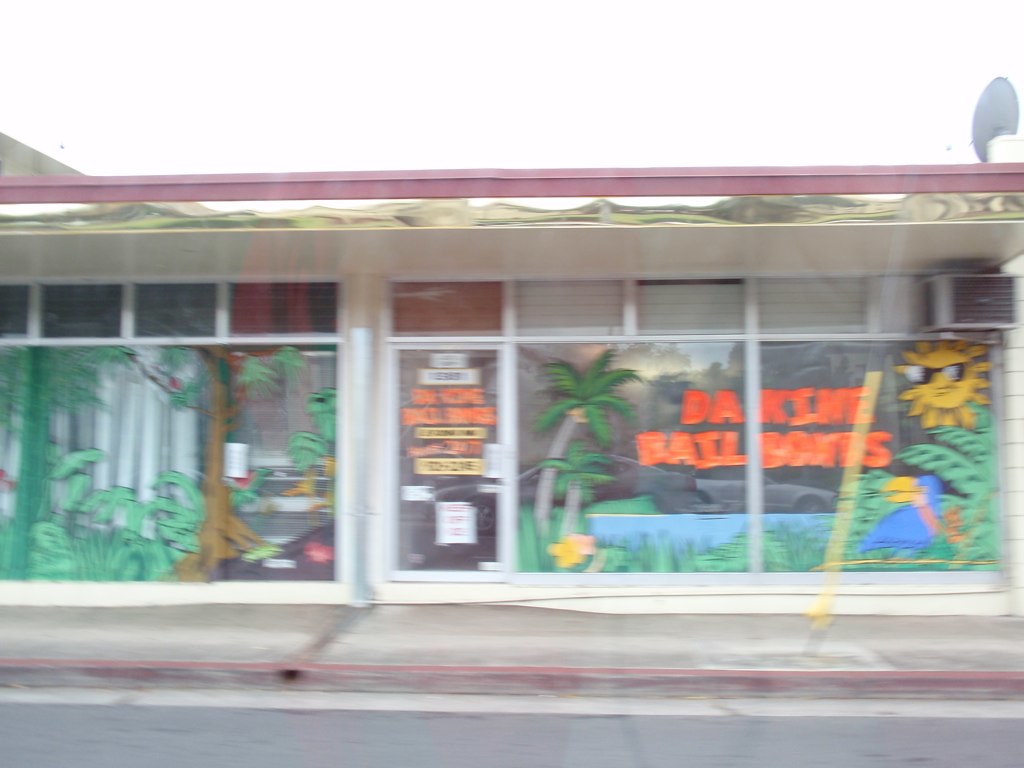The front facade of a business establishment is depicted in this image. The building features a long, flat roof with a prominent beam above it, colored a light shade of purple. The overcast sky overhead is intensely bright, casting a stark backdrop. A concrete sidewalk stretches along the front of the building, lined by a curb that appears to be painted red, leading to a gray roadway.

At the center of the building's face is a glass door, topped by another glass transom window, and flanked on either side by large glass windows. On the right side, there are two large windows each topped with smaller windows. The farthest right window has an air conditioning unit protruding from it. To the left of the door is another large window, also accompanied by smaller windows above it.

The windows are adorned with vibrant paintings; the right-side window features a cheerful painted sun sporting sunglasses, alongside palm trees. There is also orange writing that is somewhat illegible but may hint at words like "Nail," "Bail," or "Doughnuts." The left-hand side window is undecorated by any writing.